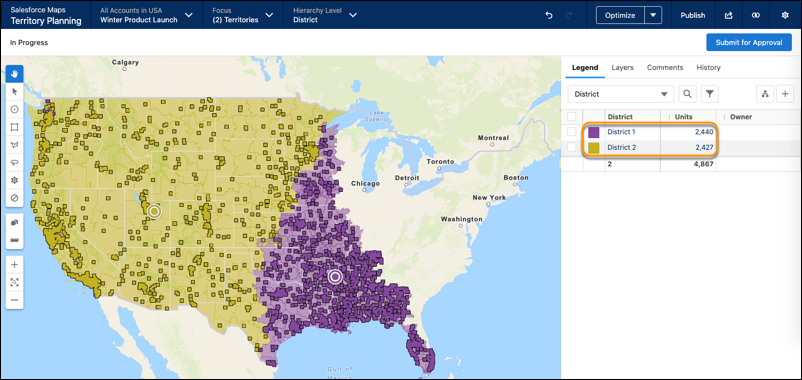The image is a screenshot of a website interface dedicated to territory planning, prominently displaying options and data related to a winter product launch. In the upper left corner, the site title "Territory Planning" is shown. The map highlights two distinct territories for the launch: one encompassing the entire western half of the United States, which is split down the middle of Texas, and another forming a purple triangle. This triangle spans from the tip of Texas up to the first Great Lake, then extends in a nearly straight line down towards Florida, covering the central portion of the United States, but notably excluding the easternmost areas.

The interface includes several navigation and command buttons such as "Optimize," "Back," "Publish," "Submit for Approval," and "Legend." The legend helps distinguish the two territories and indicates that each territory has the same number of units assigned to it. Additional options like "Layers," "Commons," and "History" are also visible, suggesting functionality for detailed geographic and historical data analysis.

The assumption is that this program facilitates regional mapping to streamline product lines, with perhaps the central district receiving a different product from the eastern district, aiding in strategic planning for the winter product launch.